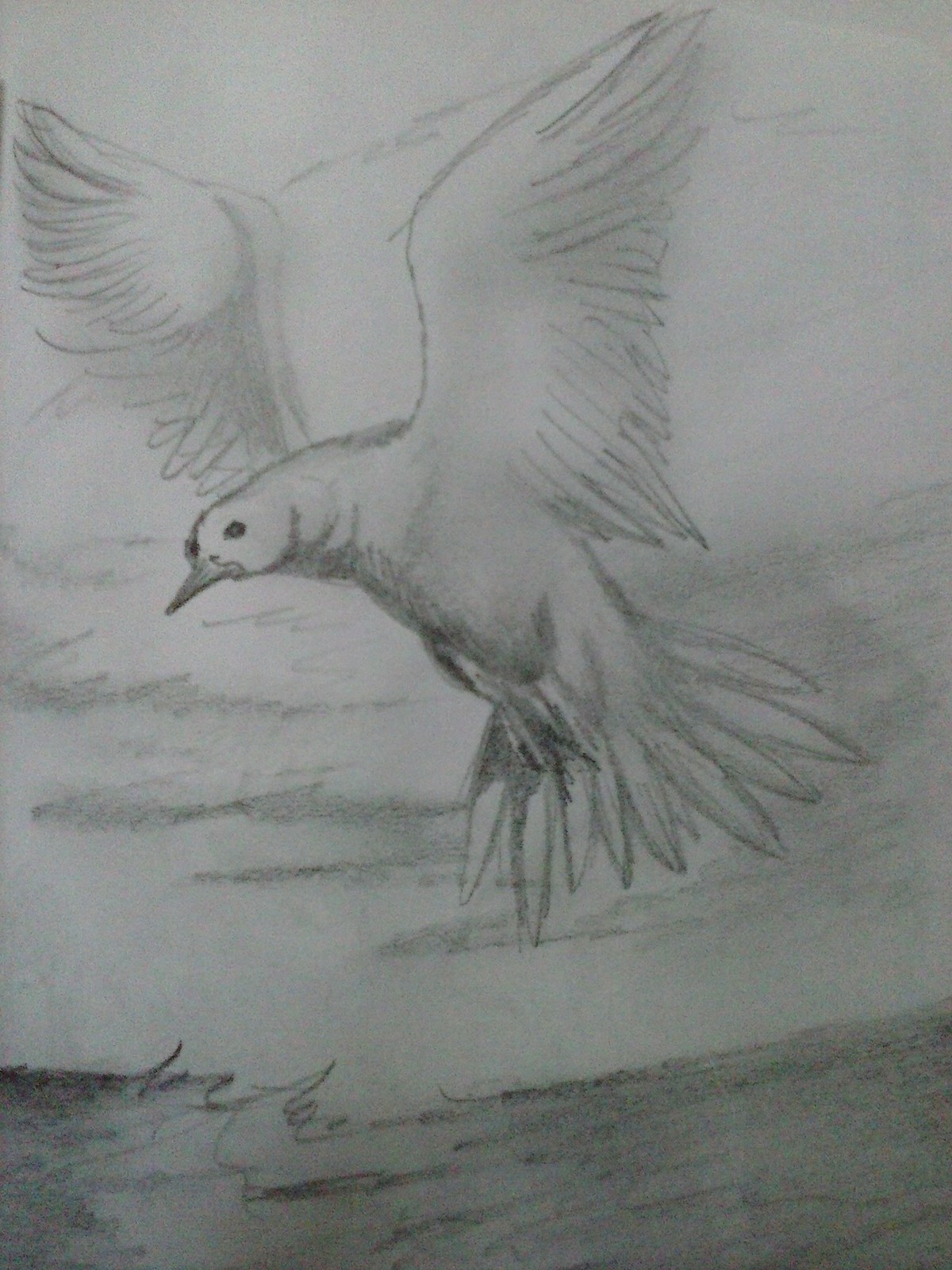This is a vertically oriented pencil sketch of a seagull in flight, created with black and gray pencil on light gray or unbleached drawing paper. The bird, which is depicted with its wings raised high and its feet tucked underneath, appears to be gliding over the water below, subtly indicated by broad, quick pencil strokes signifying movement. The seagull's body is large, with a round head, sharp pointy beak, and beady eyes positioned on either side of its head. Its tail feathers extend prominently beneath it. The detailed shading primarily focuses on the bird’s body and wings, which reveal a contrast in lightness between the left and right wing. The sky is gently illustrated with light pencil strokes suggesting clouds, blending seamlessly into the background. The overall composition features a simple yet effective shading technique that gives the otherwise monochromatic scene a sense of depth and dynamism, capturing the essence of the bird soaring high above the ocean.